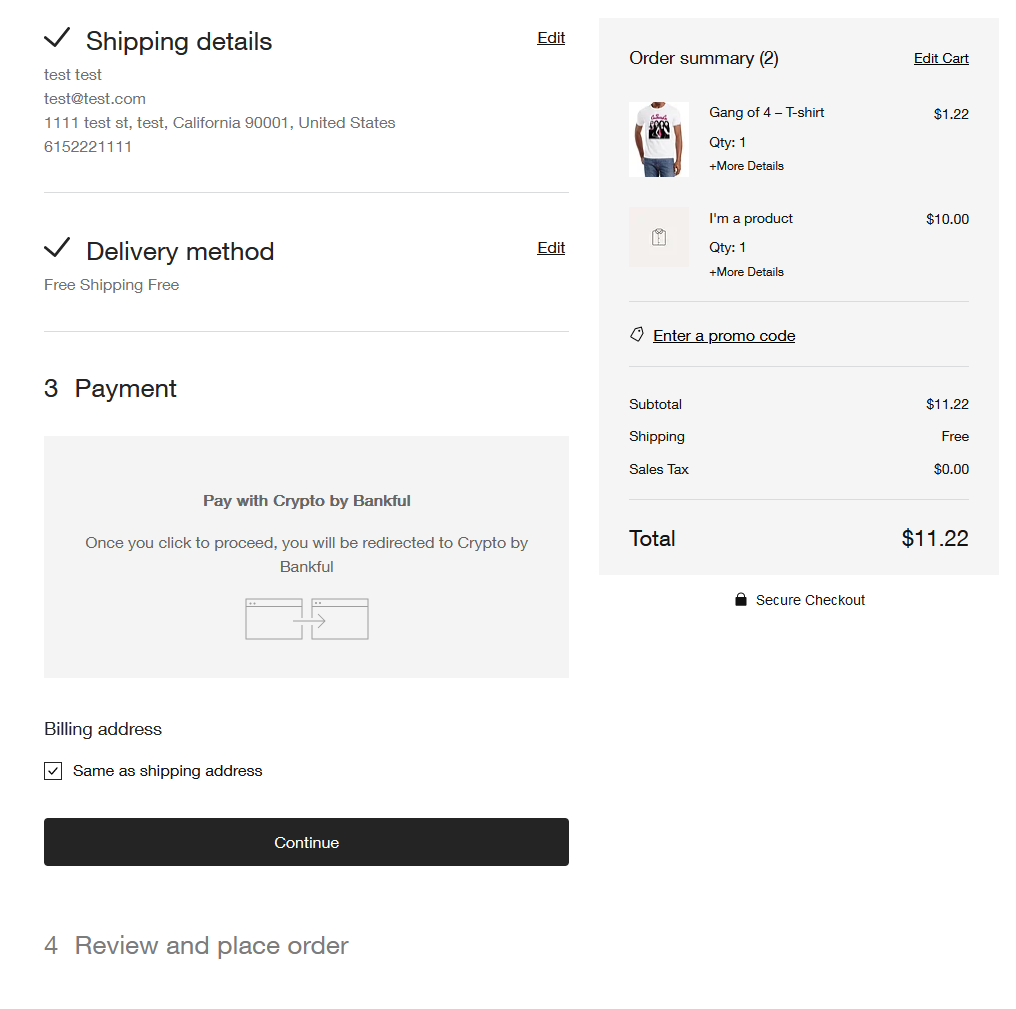This detailed caption provides a comprehensive description of an online shopping checkout page with specifics about layout, sections, labels, and icons:

---

The image depicts an online shopping checkout page with a mostly white background, except for a light blue section on the right side, starting a little less than halfway from the left to the right and then extending halfway down before returning to the right edge. 

In the upper left corner, there is a black checkmark icon with the label "Shipping Details." To its right, near the blue section, there is an "Edit" option. Below this, there are four lines of address information, followed by a horizontal line. Below the line, another black checkmark icon indicates the "Delivery Method."

On the right side of the page, within the blue section, the word "Editing" appears with smaller gray text underneath that reads "free shipping free." Beneath a gray line in this section, there is a heading labeled "Payment," followed by a light blue square containing black text that reads "Pay with Crypto by Rankful." 

Below this section, there is additional information, including two credit card icons with an arrow pointing from one to the other. To the left of this, it says "Billing Address," and beside a black checkmark, it indicates "Same as shipping address."

Near the bottom of the layout, a large black "Continue" button with white text spans the width of the page. Below this are the options for "Review and Place Order."

In the blue portion, towards the top left, the label "Order Summary" is displayed, with the number "2" in parentheses. On the right side of this section, an underlined "Edit Cart" option appears. The section includes a picture of a white t-shirt and blue jeans on the left side, with three lines of information and the price on the right side. 

There is an empty square with three lines of information and a price on the right side. Beneath this, a promo code entry area displays "Enter a Promo Code," followed by details about the subtotal, sales tax, and total cost, with corresponding amounts on the right side.